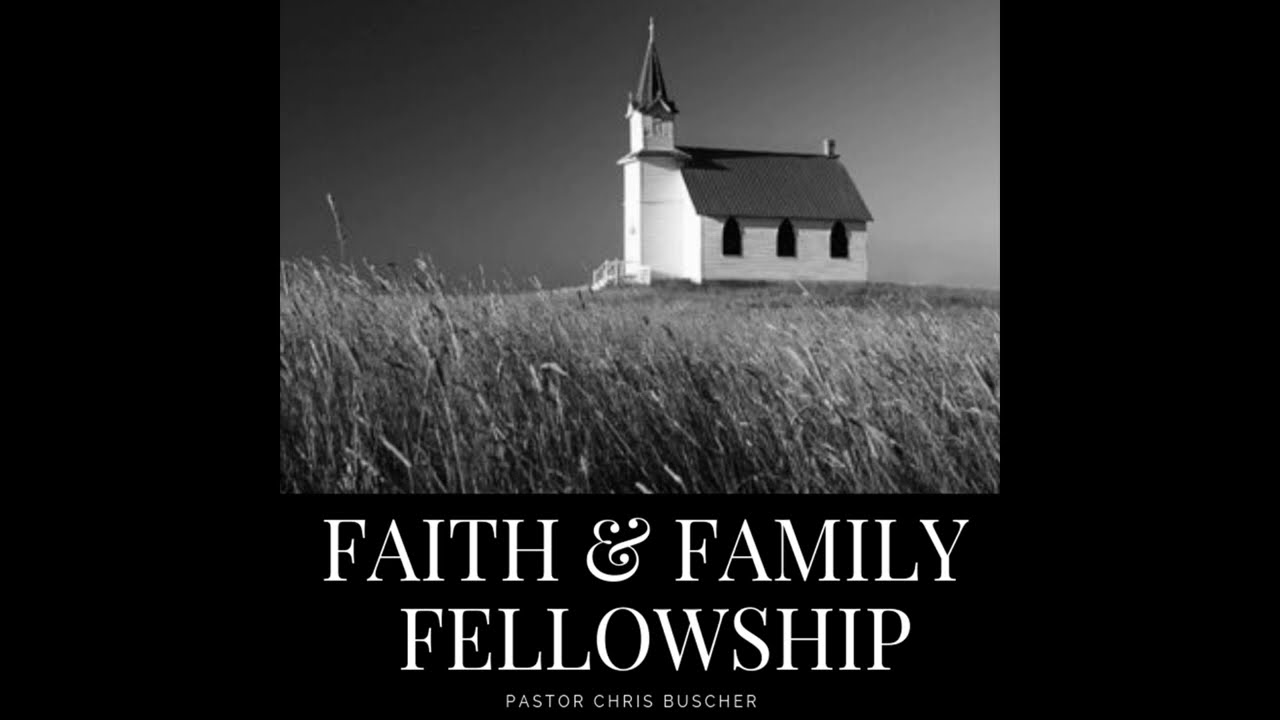The grayscale collage features a small town church prominently positioned against a black background that encircles the left, right, and bottom parts of the image. In the center and extending to the top, the black-and-white photograph captures the church amidst a sweeping field of wheat or tall grassy weeds, reminiscent of a scene from "Little House on the Prairie." The church itself displays classic architecture with a white wooden exterior, a medium-colored dark shingled roof, and a steeple tower rising above. On the side of the building facing the camera, there are three evenly spaced windows. Leading up to the entrance are some stairs. Beneath this clear and detailed visual, white text reads "Faith and Family Fellowship," with the "and" symbol artistically transformed into a heart shape. Smaller text below this headline identifies the affiliated individual as "Pastor Chris Buscher."